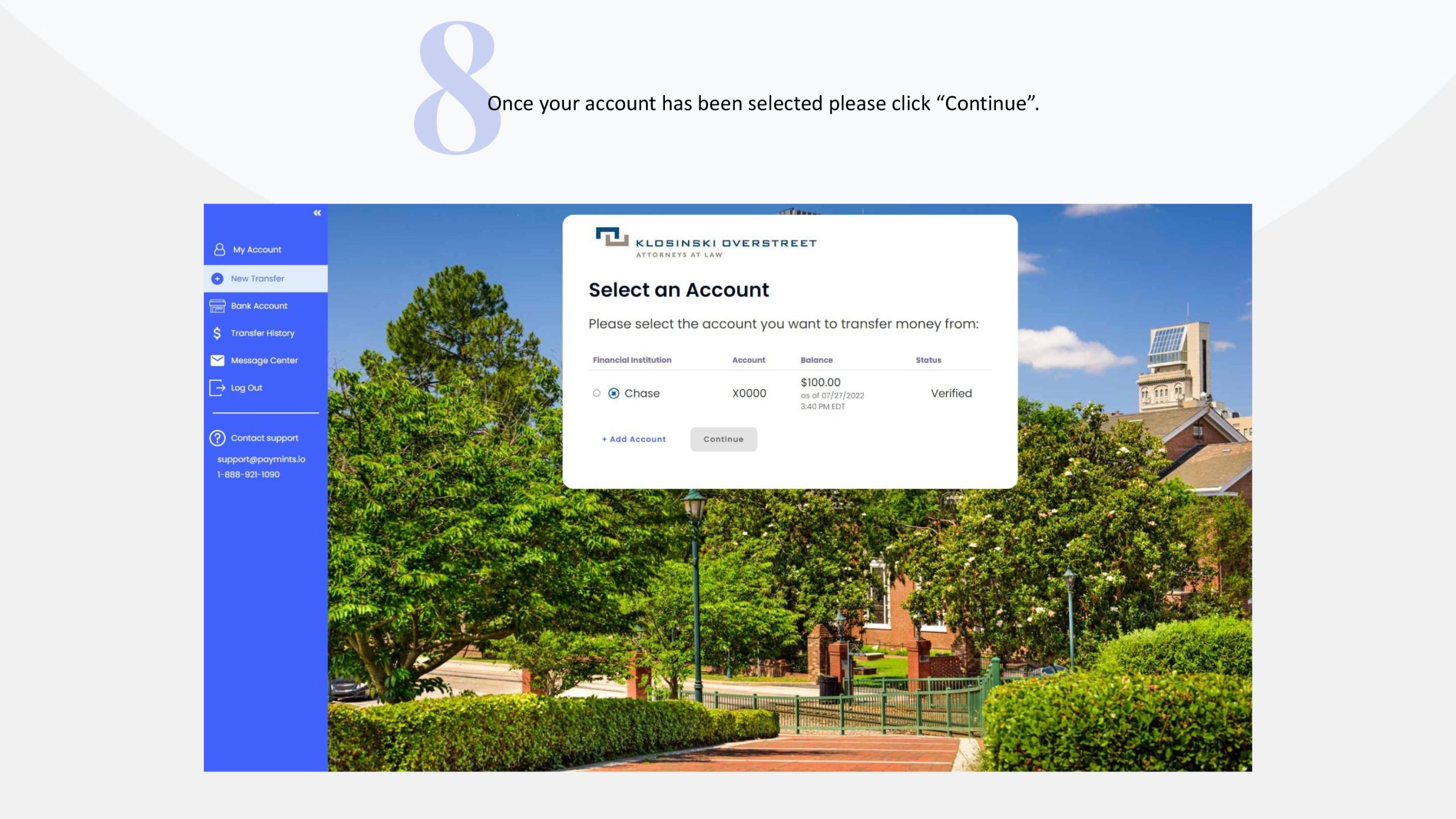This rectangular image is a detailed screenshot primarily displaying a user interface for account management under the banner "Klosinski Overstreet Attorneys at Law." The interface includes a white rectangular box superimposed over a scenic background photograph featuring a lush, treed area and a prominent red brick building.

Within the white box, the interface prompts the user to "Select an account." Below this prompt, users can choose the account from which they wish to transfer money. The details displayed include an example account with a balance of $100, dated July 27, 2022, at 3:40 p.m. Eastern Time, associated with the financial institution Chase.

The left side of the image features a vertically-oriented, blue sidebar with navigation options listed as follows from top to bottom: "My Account," "New Transfer" (highlighted), "Bank Account," "Transfer History" (accompanied by a dollar sign icon), "Message Center," "Log Out," and "Contact Support at support.payments.io."

This detailed interface layout effectively guides the user through the process of managing financial transactions, enveloped by a visually appealing background setting.